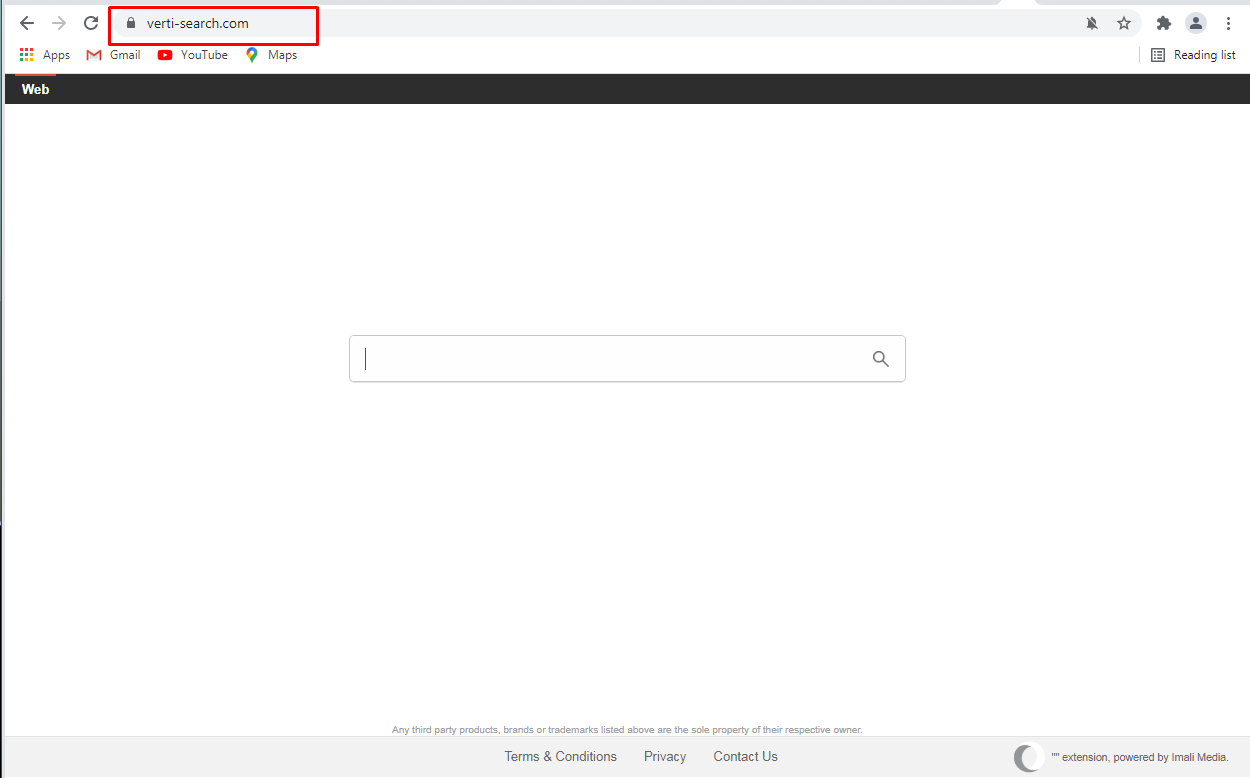### Detailed Image Caption

The image depicts a screenshot of a website with a white background. In the top left corner, there are navigation arrows with a bolded left-pointing arrow, followed by a refresh button enclosed in a rectangular box with a red border. Adjacent to this box is a lock icon next to the URL, which reads "VERTI-search.com". 

On the top right of the screenshot, there is a row of icons including a face icon with a line through it, a star, a puzzle piece, a placeholder for a user thumbnail, and three vertical dots. Below this, on the far left, there is the Google Apps icon followed by the Google logo, and links labeled "Apps," "Gmail," "YouTube," and "Maps" which also includes a Maps pin icon. On the far right of this line, it reads "Reading List."

On the line below, a black rectangular box stretches across the page with the word "web" written in white text. Dominating the center of the page is a prominent search bar accompanied by a search icon. At the bottom of the page, there are links for "Disclaimer," "Terms and Conditions," "Privacy," and "Contact Us." In the bottom right corner is the company's logo.

This layout combines various navigation and utility features common to web browser interfaces, arranged in a clean, user-friendly design.